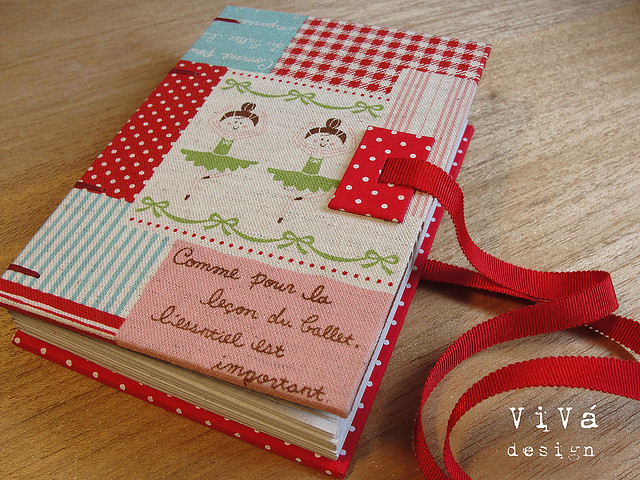The image is a detailed photograph of a closed, colorful book lying diagonally at the center of a light brown, wooden table. The setting appears to be indoors and illuminated by natural daylight. The book itself features a cloth covering adorned with an array of colors including brown, light blue, white, red, green, tan, and pink. 

Prominently displayed on the cover are two cartoon-style ballerinas with black hair in buns, white faces with small dots for eyes, and upturned mouths. They are dressed in green shirts. A red ribbon can be seen emerging from the book near where the pages would open, likely for tying the book closed. The cover also includes a red and white checkered portion at the top right, and a red rectangle with white dots running down the spine.

A green ribbon crosses the center of the cover on the bottom right over a pink background, displaying brown text in French: "Comme por la leçon de ballet. L'essencial est important." In the lower right corner, the brand "Viva Design" is printed in white lettering.